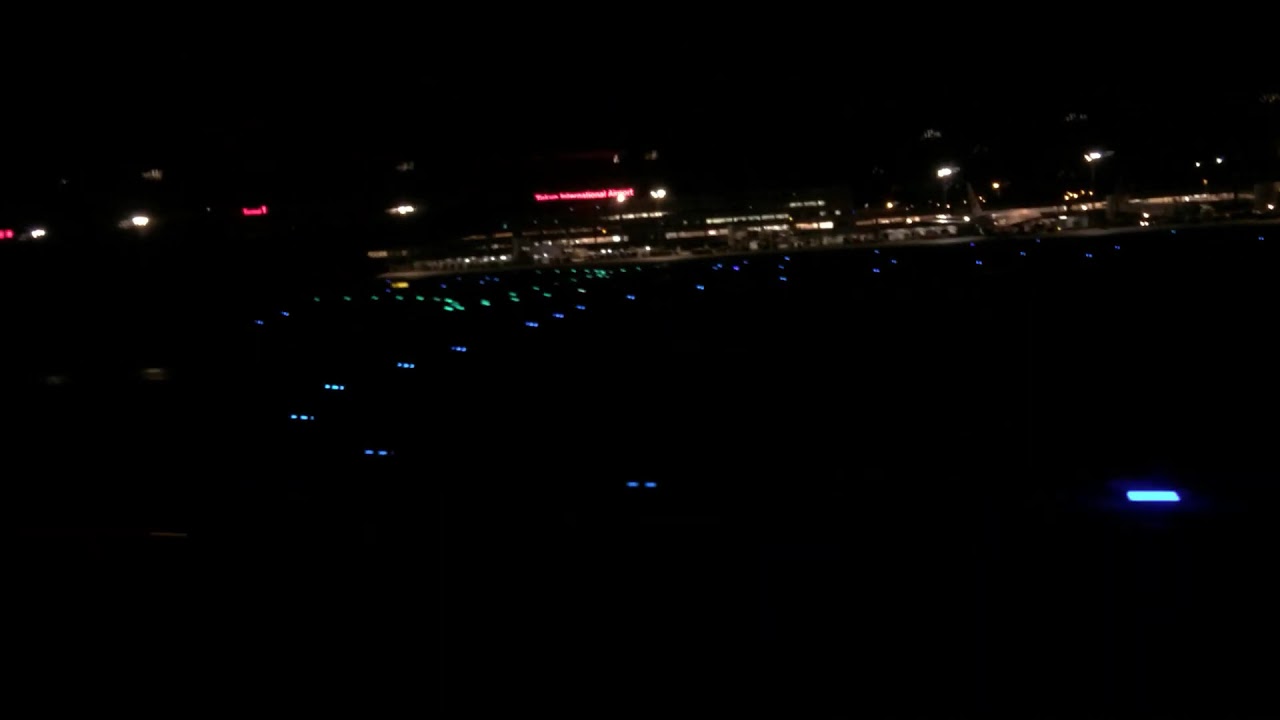The image captures a nighttime scene, predominantly dark with scattered lights in various colors. The most visible lights are blue, green, orange, and yellow, emanating from the lower right side and rising diagonally towards the upper right. These lights are likely part of an airport runway, aiding pilots during takeoff or landing. In the middle and upper portions of the image, there's a distant, well-illuminated building with an interior that suggests glass-fronted structures, strongly lit from within. Despite the generally pixelated and blurry quality of the image, caused by it being a screenshot from a video, there are possibly cars or people around, though it's difficult to discern due to the darkness and pixellation. Additionally, above the illuminated building, there's a row of lights in white and pink. The overarching darkness of the image renders much of the scene indistinguishable, but the bright dots of light punctuate the otherwise black canvas, hinting at an active, functioning airport environment.